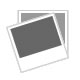The image is an advertisement showcasing a heavy yellow excavator situated near a river, with industrial buildings and a cityscape in the distant background under a blue sky dotted with wispy clouds. The excavator is positioned on a dock-like platform alongside two large steel beams and an additional mast. There's prominent text on the bottom half of the image that appears to be a review, stating, "Look forward to future business with this seller. Thanks again, excels in customer service, super fast shipping!!" The logo of the company, identified as Stevens Blake Parts, is also present, though parts of it, specifically the yellow text, are difficult to read.